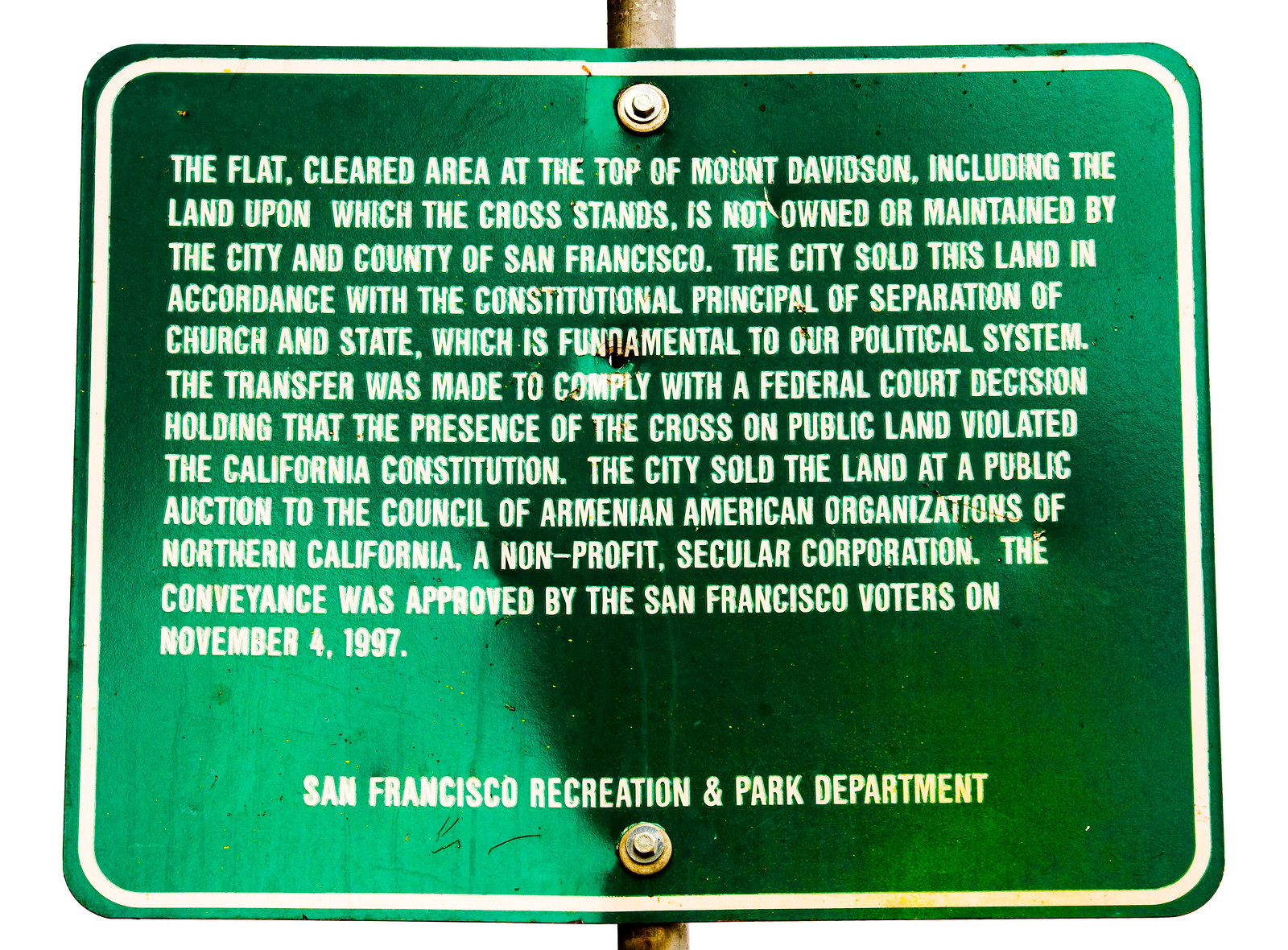This wide, rectangular image captures a bright green, metal government sign affixed to an old, rusty metal pole with two visible bolts securing it. The sign, which is slightly shinier and more reflective on the bottom left side and top middle, features rounded corners and a white border tracing its outline. In thick, all-caps white letters, the detailed text informs that the flat, cleared area at the top of Mount Davidson, including the land upon which the cross stands, is not owned or maintained by the City and County of San Francisco. It goes on to explain that the city sold this land in accordance with the constitutional principle of separation of church and state to comply with a federal court decision that found the cross's presence on public land violated the California constitution. The land was sold at a public auction to the Council of Armenian American Organizations of Northern California, a non-profit secular corporation, with the conveyance approved by San Francisco voters on November 4, 1997. The bottom of the sign indicates it is from the San Francisco Recreation and Park Department.